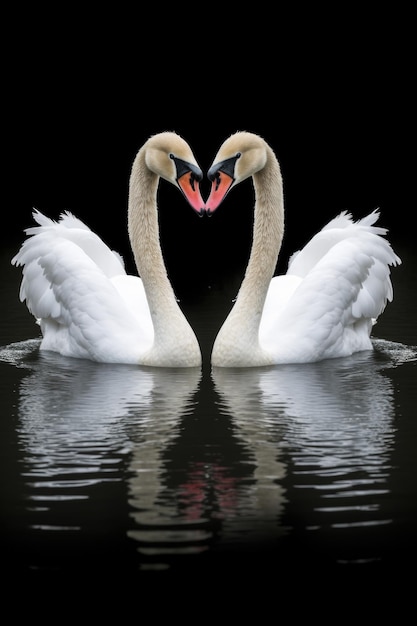In this captivating photograph, we see two elegant swans gracefully positioned in tranquil waters. The swans' heads come together, forming a heart shape that exudes a tender and romantic aura. The background is a deep, flat black, creating a striking contrast that accentuates the purity of the scene. The lower part of the image also fades into black, blending into the water's grayish hue. This gray water gently reflects the swans, with white ripples adding a touch of texture and depth.

The swans showcase their pristine white feathers, which glow brilliantly against the dark backdrop. Their wings are subtly elevated, giving them a graceful and majestic appearance. The swans' necks, slightly off-white, curve elegantly upward before their heads tilt downward. The birds' bills are vivid orange near the tips, transitioning to a darker black near the eyes, creating a striking visual contrast. The swans touch bills tenderly, further emphasizing the heart shape they form together, making this image a truly enchanting capture of avian affection.